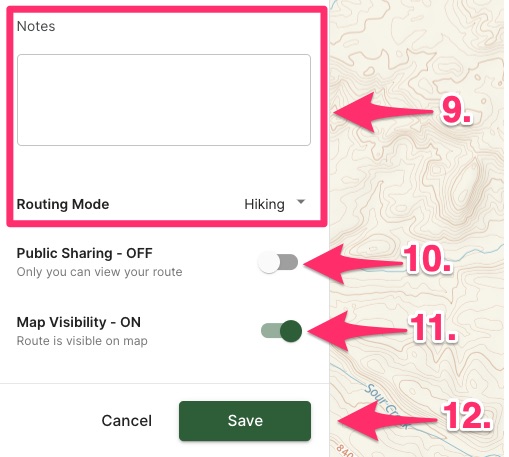This image is a detailed screenshot of a map interface with annotations and various options highlighted. On the far right, occupying about one-third of the image from top to bottom, is a map displaying a location marked by the words "Sauer Creek" in light blue text. An arrow partially obscures the word "Creek," but the destination appears to be Sauer Creek.

The screenshot also features four arrows and their respective numbers, all in pink, indicating different elements of the interface:

1. The number 9, accompanied by a pink arrow, points to the left towards a framed section labeled "Option Notes." Within this frame, there is a section at the bottom labeled "Routing Mode," with "Hiking" selected from a drop-down menu.
2. The number 10, also with a pink arrow pointing left, indicates the "Public Sharing" option, which is currently toggled off, signifying that only the user can view the route.
3. The number 11, again with a pink arrow pointing left, targets the "Map Visibility" toggle, which is switched on (displayed in green), meaning that the route is visible on the map.
4. The number 12, with another pink arrow pointing left, highlights the "Save" button. This is shown next to a "Cancel" button, with "Save" written in white text on a green button.

Overall, the image provides a comprehensive view of the map's interface, focusing on the location "Sauer Creek" and various important settings and options available to the user.